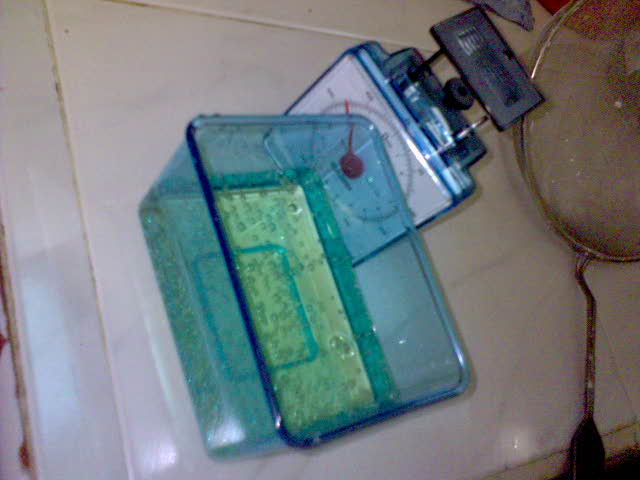In this detailed color photograph taken from above, we see a laboratory setting with a fairly dirty white tabletop. Central to the image is a scale, featuring a white dial with black lettering and a red needle, encased in a blue frame, with a silver, steel platform above it. In front of the scale rests a plastic dish, which is semi-transparent blue with a yellow bottom and appears to fit onto the scale's platform. The dish contains a thick, almost clear liquid with a slight yellowish tint. To the right of the scale is a metal strainer, characterized by its round mesh form, long silver handle, and a black rubberized end. The setup also includes what looks like a metal pot, suggesting this simple yet functional laboratory equipment is being used for an experiment.